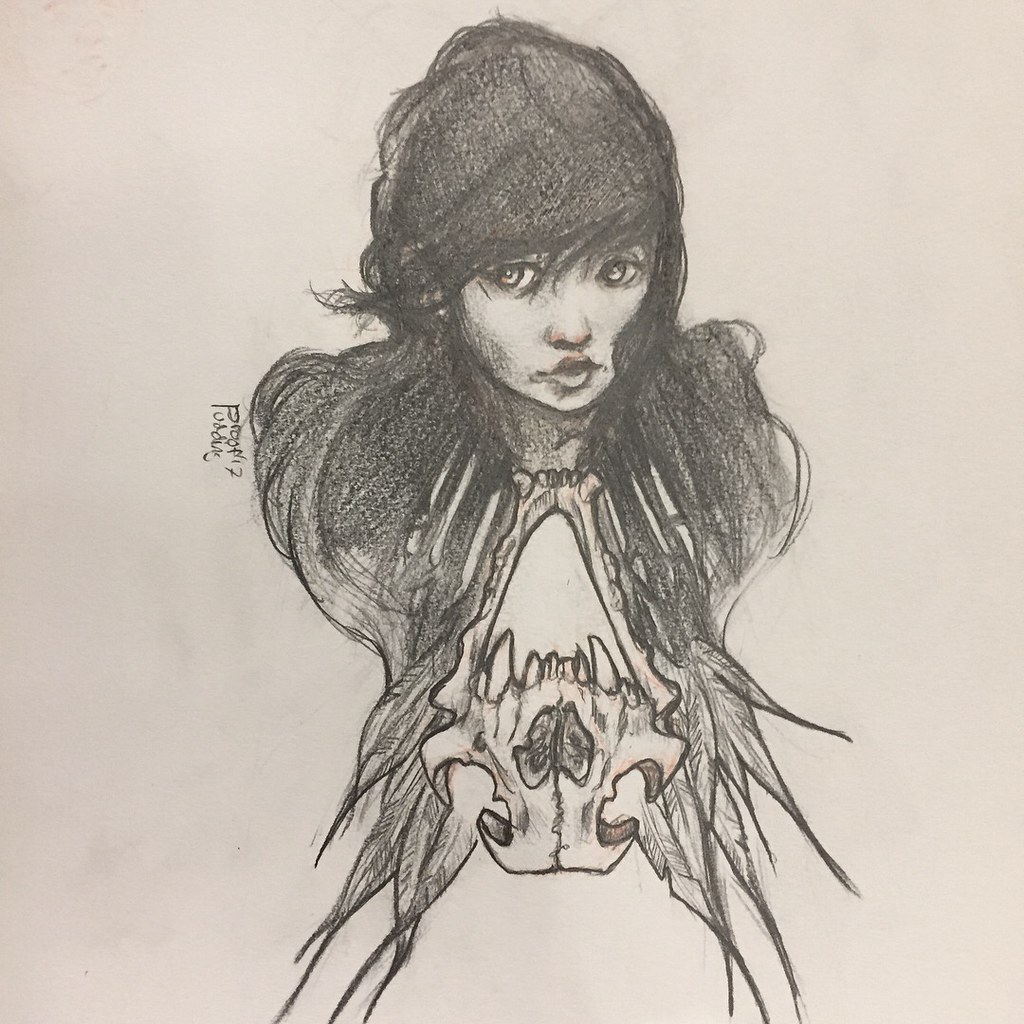This is an intricately detailed pencil sketch of a young woman with dark, flowing hair that cascades over her shoulders. Her eyes are wide open, gazing to the left side of the image, partially covered by long, shaggy bangs. The sketch captures just the head and shoulders of the woman. Below her head, there is an upside-down animal skull, resembling that of a tiger, with sharp, pointy teeth and a noticeable broken piece around the eyes. The jaw of the skull aligns precisely with her own jaw. Gray feathers, three or four on each side, fan out from the bottom of the skull, adding a dramatic flair. A small signature from the artist is discreetly placed to the left of the woman's head, blending in with the background. The entire composition exudes a hauntingly beautiful and surreal quality, brought to life through the meticulous pencil work.